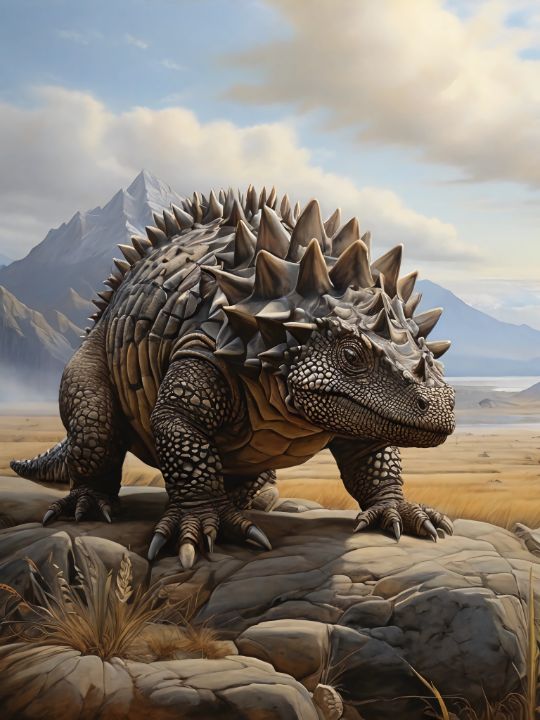This detailed image features a digitally reconstructed ankylosaurus, depicted in a prehistoric North American landscape. The ankylosaurus stands prominently on a beige rock mound with some patches of brown grass. This formidable creature is portrayed with a body covered in tan and brown scales, and an array of spikes and horns that extend from its head along its back to its tail, resembling a heavily armored lizard. Its anatomy includes four toes on each front foot and three on each back foot, and its underside bears a texture similar to a turtle’s belly. The creature is positioned on all fours, seemingly walking towards the viewer while staring directly at the camera. The background features an expansive, dry landscape with wheat fields, rocky plains, and a mix of land and water bodies. This scene is framed by steep, misty mountains capped with peaks, under an overcast sky dotted with puffy white and gray clouds, allowing occasional glimpses of blue sky. The overall atmosphere is one of ancient earth, vividly recreated to showcase both the majestic ankylosaurus and its natural habitat from millions of years ago.